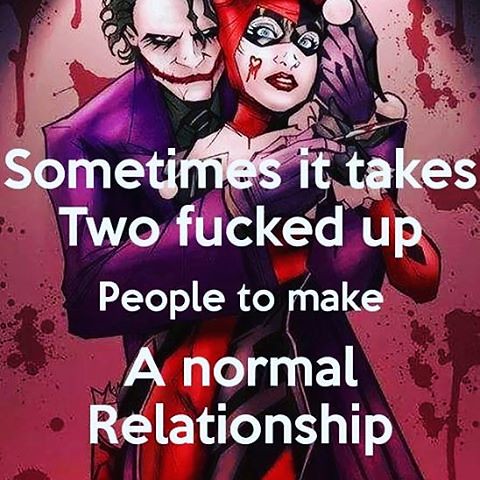In this comic book drawing, two iconic characters, the Joker and Harley Quinn, are depicted with vivid, intense details. The image features the Joker wearing a purple suit, a green shirt underneath, and a black and white tie, holding a knife in his right hand. His face is painted white with red accents, showcasing his menacing appearance. Harley Quinn, dressed in a distinctive red and black jumpsuit with black facial markings and pale skin, appears to be in distress as she is held from behind by the Joker. The background is a striking whitish-red hue, splattered with what appears to be blood, enhancing the dramatic tension of the scene. White text overlays the image, stating, "Sometimes it takes two fucked up people to make a normal relationship," further emphasizing the tumultuous and dark nature of their relationship. The art style is gritty, capturing the chaotic and dangerous essence of these two infamous characters.